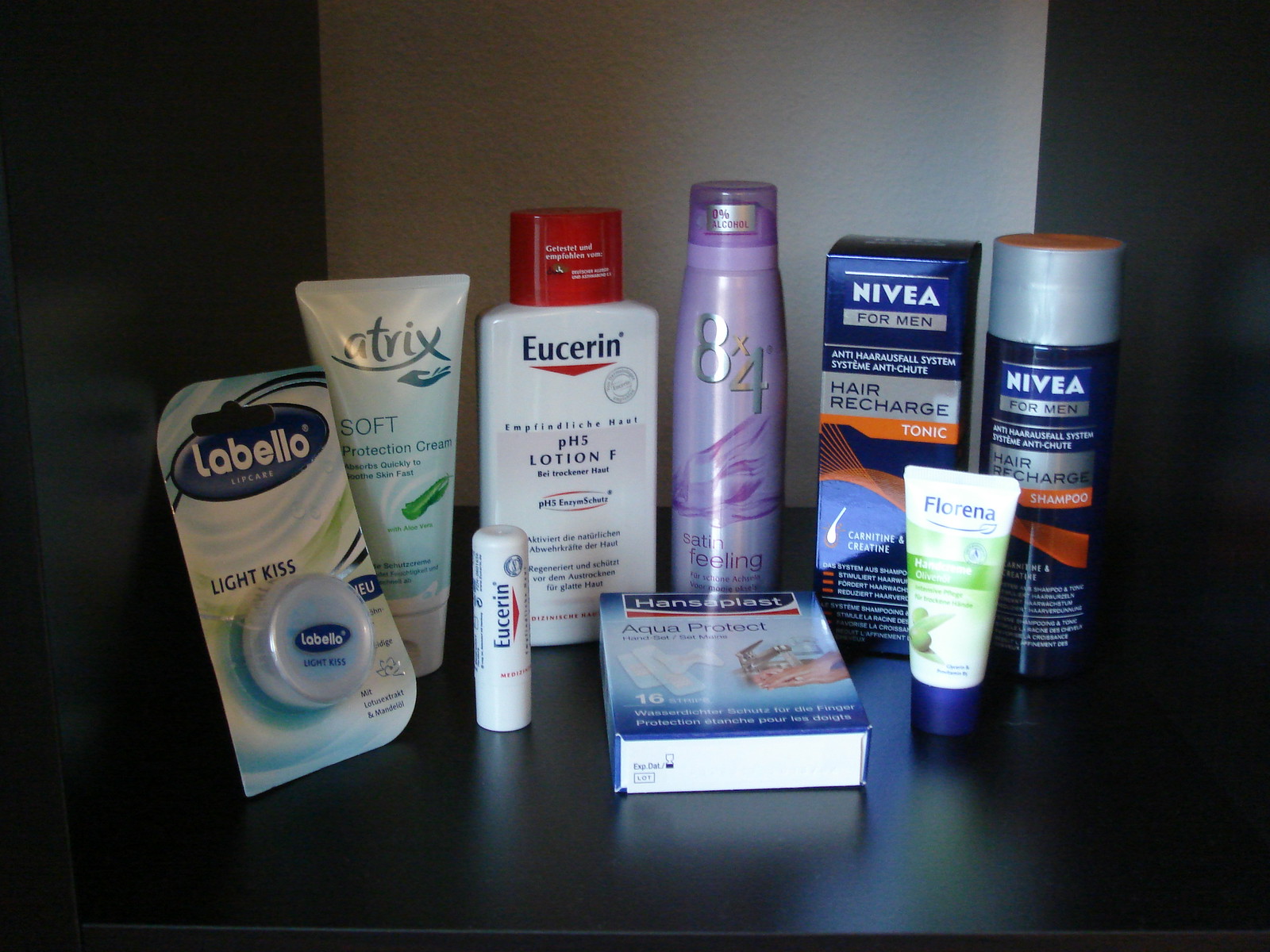In the image, there is a display against a black background with a shimmery black countertop. In the middle of the image, there's a white backdrop. On the left side, there is a round blue container with white letters spelling "Labello" featuring the words "Light Kiss" in blue letters next to it. Beside it, there is a product called Atrix with a blue container and white cap, labeled "Soft Protection Cream."

Next to Atrix, there is a white bottle with a red cap that reads "Eucerin" in dark blue letters with a red arrow pointing downwards. The label also mentions "PH5 Lotion F" on a light pink background. Adjacent to this is a purple bottle with the number "84" and the phrase "Satin Feeling" below it on what appears to be a satin sheet.

Next in line is a blue box with "Nivea" in white letters, next to a gray box with black writing labeled "For Men." This box is for a Hair Recharge Tonic featuring white letters and an orange highlight. Following this box is a gray bottle with an orange cap, blue background, and white letters saying "Nivea For Men Hair Recharge," which presumably came from the aforementioned box.

Further on, there is a small white plastic squeeze bottle from "Florina" with a green banner. Next to it is a box labeled "Hansaplast" for Acroprotect, probably containing bandages. The box has a blue top section, a red stripe under the title, and a white bottom section.

Lastly, there is another product from Eucerin with white packaging, a red arrow beneath the text, and black lettering.